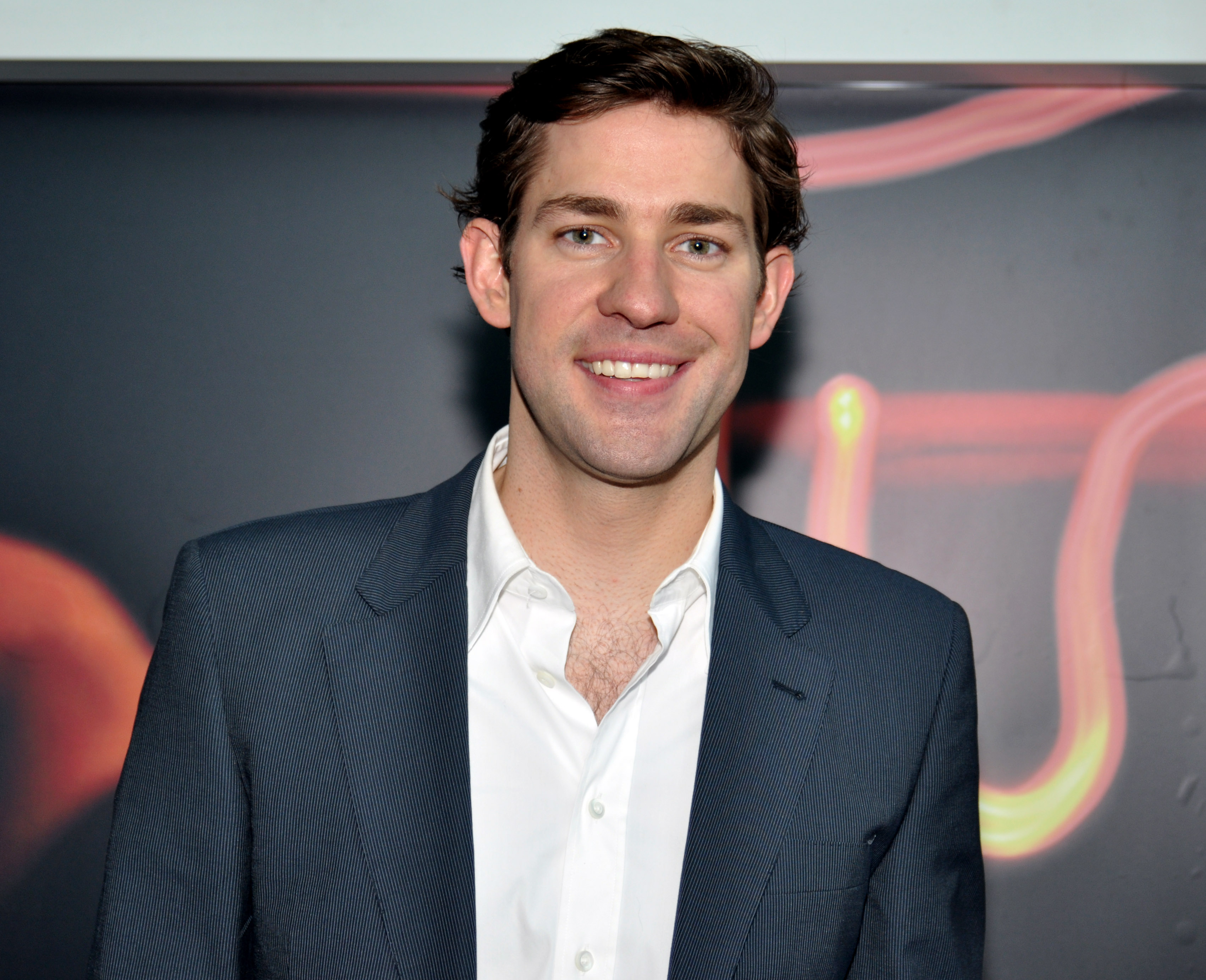This is a professionally taken photograph of John Krasinski, renowned for his role in the American version of 'The Office.' He stands centered in the image, captured from his midriff up. John is smiling warmly and making eye contact with the camera, exuding a friendly demeanor. He is dressed in a smart, medium-dark gray blazer paired with a white shirt that's unbuttoned at the top, revealing a hint of his chest hair. His dark hair is neatly styled, and he has dark brown eyes, pronounced dark brown eyebrows, and very pink lips complementing his smile. Though his teeth are a bit stained, his overall appearance is polished and approachable. His slightly crooked nose adds a charming touch to his look. The background features a gray base with curves and bands of light, adorned with colors including peach, black, red, orange, and yellow, giving the impression of a red carpet event or another high-profile setting.